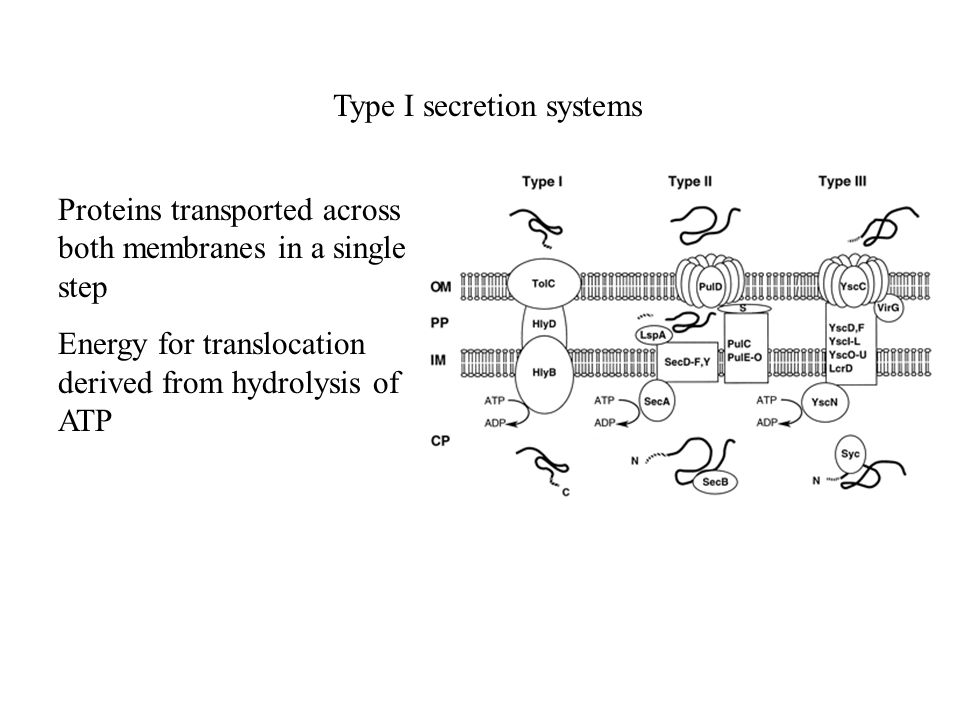This black and white diagram, likely extracted from a textbook, details the Type 1 secretion systems. The header at the top states "Type 1 secretion systems," followed by the information on the left which reads, "Proteins are transported across both membranes in a single step," and "Energy for translocation is derived from hydrolysis of ATP." The right side of the page features a series of illustrated diagrams, each labeled with Type 1, Type 2, and Type 3 at the top. These diagrams include round circles, squiggly lines, arrows, and various labels such as "OMPPIM" and "CP," visually representing the biochemical processes described in the text.